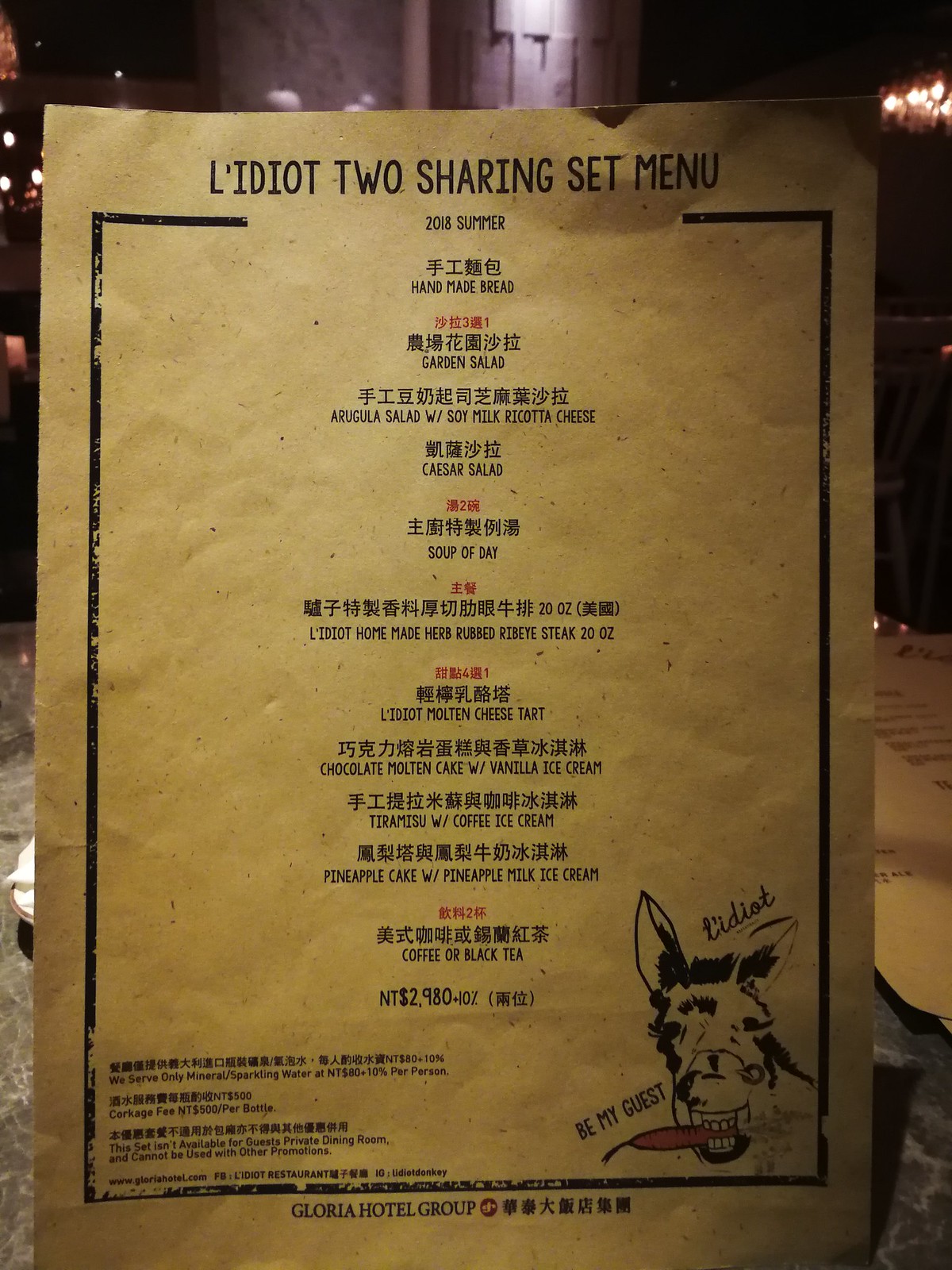This vibrant color photograph, captured in portrait mode, depicts an indoor shot of a slightly crumpled and wrinkled menu. The menu, printed on yellowish-tan parchment-like paper, exudes a rustic charm. At the bottom right corner of the menu, a whimsical drawing of a smiling donkey, cheerfully holding a carrot between its teeth, adds a playful touch. The donkey is accompanied by a speech bubble that reads, "Be my guest."

The title of the menu reads "El Idiot 2 Sharing Set Menu" in bold typography, with "2018 Summer" inscribed underneath in smaller typeface. The menu items are listed in both Asian and English characters, with some items highlighted by red Asian characters above them. 

The English items are presented in the following order:
1. Homemade Bread
2. Garden Salad
3. Arugula Salad with Soy Milk Ricotta Cheese
4. Caesar Salad
5. Soup of the Day
6. El Idiot Homemade Herb-Rubbed Ribeye Steak (20 ounces)
7. El Idiot Molten Cheese Tart
8. Chocolate Molten Cake with Vanilla Ice Cream
9. Tiramisu with Coffee Ice Cream
10. Pineapple Cake with Pineapple Milk Ice Cream
11. Coffee or Black Tea

The bottom of the menu features the insignia "Gloria Hotel Group" followed by additional Asian characters. This detailed menu provides a glimpse into an indulgent dining experience curated for the summer of 2018.